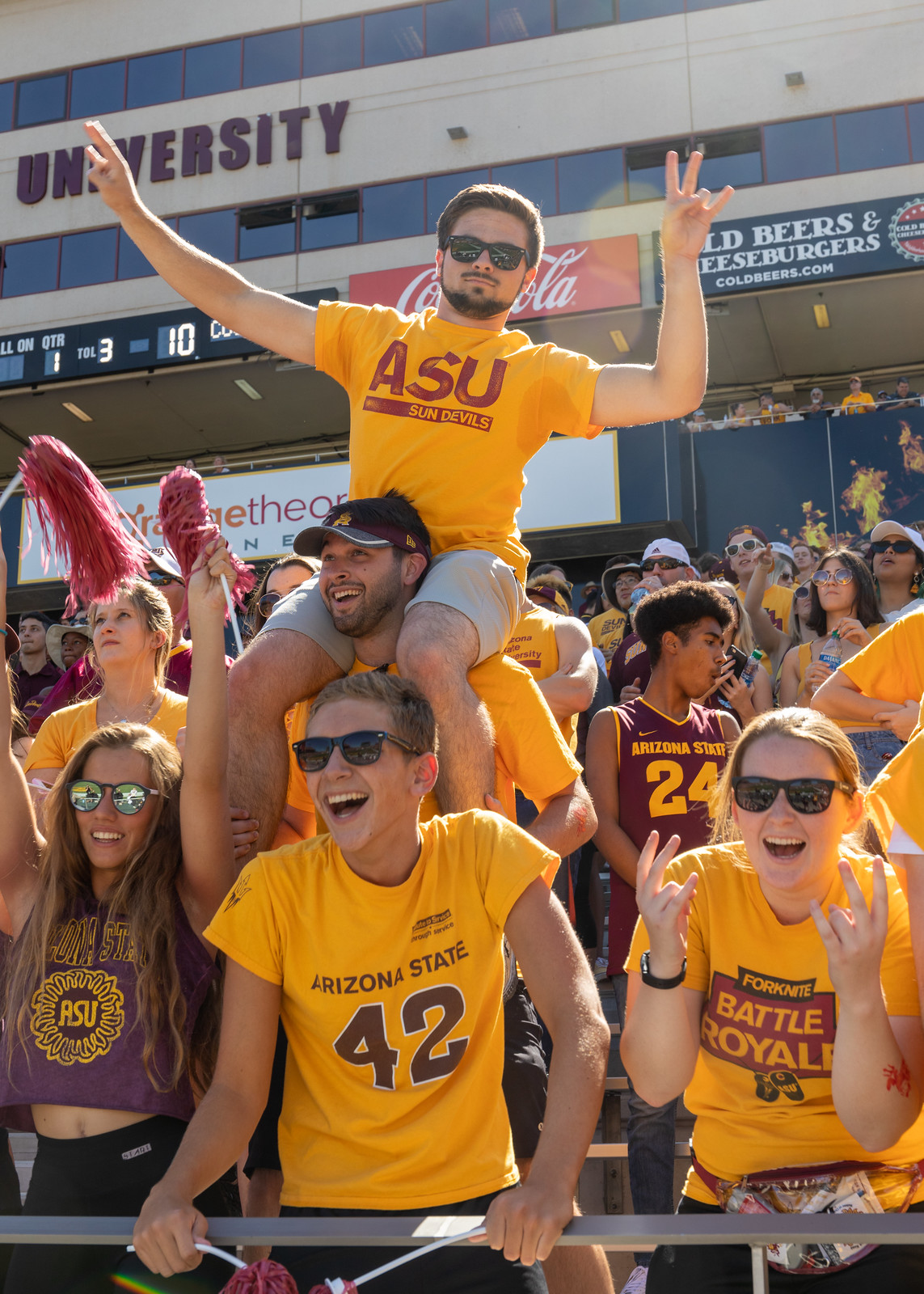In this vibrant scene from an Arizona State University football game, enthusiastic fans decked out in yellow and red are gathered, creating a lively sea of school spirit. Many of the fans, primarily appearing to be university students aged between 18 to 22, wear t-shirts emblazoned with "Arizona State," "ASU," and player numbers like 42 and 24. One particularly enthusiastic fan in the second row hoists another person onto his shoulders, much to the likely annoyance of those seated behind. The atmosphere is charged, with fans cheering, shouting, and some waving pom-poms, despite not being official cheerleaders. In the background, the scoreboard indicates that one team, presumably Colorado, has 10 points in the first quarter with three timeouts left. Advertisements for Coca-Cola, cold beers and cheeseburgers, and Orange Theory lend a commercial backdrop to the electrifying moment. The fans' attire of short sleeves and shorts, combined with the bright and sunny weather, hint at a typically warm Arizona day.